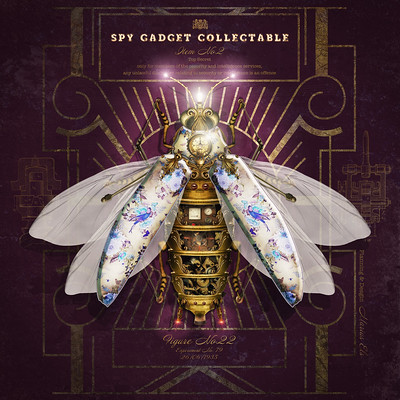The image depicts a highly detailed, stylized mechanical wasp or bumblebee set against a purplish background with gold patterns. The title "Spy Gadget Collectible" is prominently displayed in gold lettering at the top. The bee's body is primarily golden and features four visible compartments, each containing intricate clockwork mechanisms, gadgets, and dials. Near the head of the bee, a visible watch-like dial adds to the mechanical aesthetic. The bee has six wings in total; two feature vibrant purplish-bluish designs, while the remaining wings are translucent. The antennae and the tip of the mouth are illuminated, adding a touch of light to the intricate metalwork. The background also includes additional text that might suggest "figure number 22" or a similar designation, contributing to the impression that this is part of a collectible series.